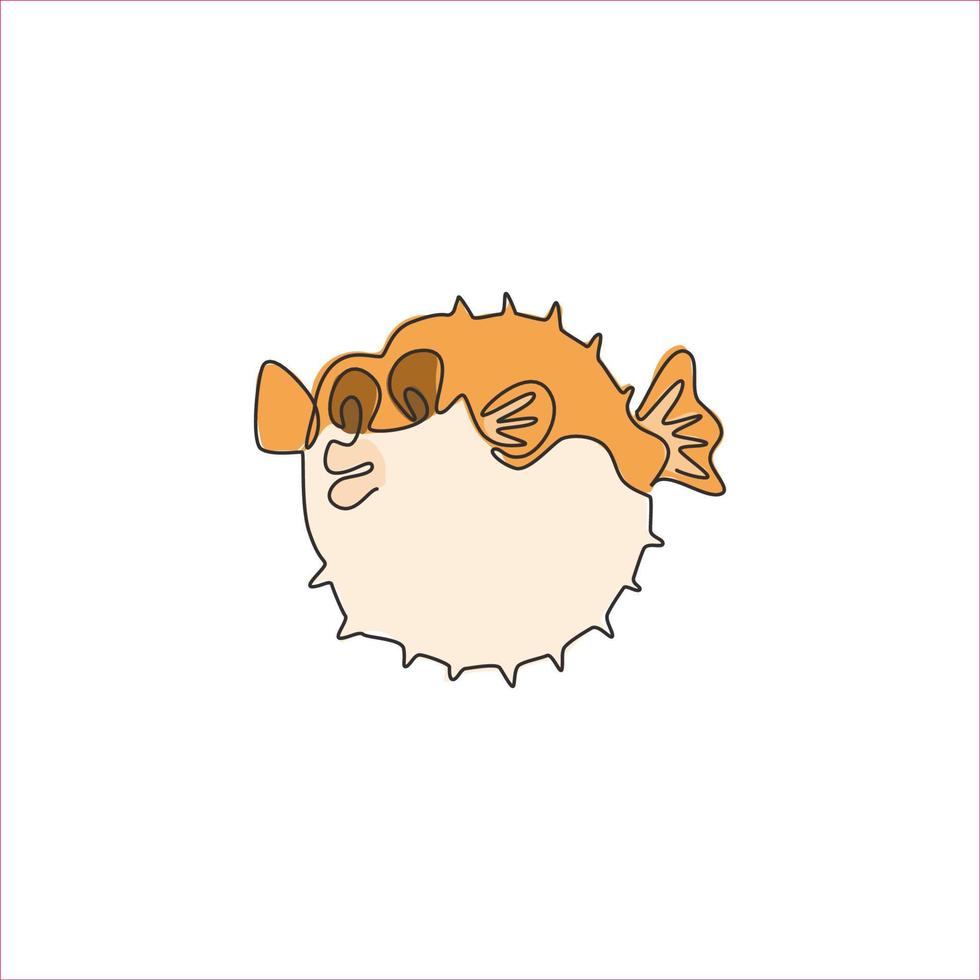The image portrays a square cartoon drawing of a jovial pufferfish centered on a stark white background, accented with a thin light black trim. The pufferfish, depicted in a cutesy art style, is fully puffed up in its defensive state, resembling a perfect circle with protruding fins. Its top half, including the fins and tail, is shaded in a light orange hue, while the bottom half is a soft tan or off-white color. The pufferfish's closed eyes are dark brown with lighter brown surrounding them, adding to its blissful expression. Its mouth is whimsically pursed into two prominent lips. The fins are orange, with the closer fin featuring three off-white segments, akin to fingers, a design mirrored in the tail. Decorative spikes adorn the top and bottom edges of its body, enhancing its vibrant and playful appearance.